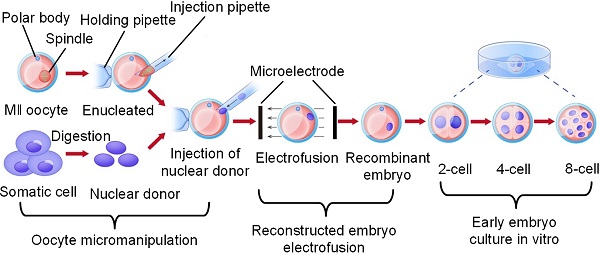The image depicts a detailed scientific chart illustrating the steps involved in a cell manipulation process, possibly related to embryonic development or cloning. At the top, it highlights key elements such as the "injection pipette" and "holding pipette," with arrows indicating their respective positions. The chart features labeled parts including the "polar body," "spindle," and "somatic cell nuclear donor." The process appears to follow a flowchart format, starting with initial steps involving the manipulation of these cells.

The cells are color-coded for clarity, with pink circles representing different stages of the embryo, progressing from "two-cell," "four-cell," to "eight-cell." Another section in purple shows additional cells labeled "somatic cell," which are involved in the nuclear donor process. Arrows guide the viewer through the stages of "microelectrode electrofusion," leading to a "reconstructed embryo."

Further steps show the development of the embryo, labeled as "recombinant embryo," "early embryo," and include stages of "early embryo culture in vitro." Underneath these stages, the chart references "digestion" and "octet micro manipulation," indicating various techniques involved in the process. Overall, the image serves as an instructional guide, detailing each step from the injection of the nuclear donor to the cultivation of the early embryo culture.